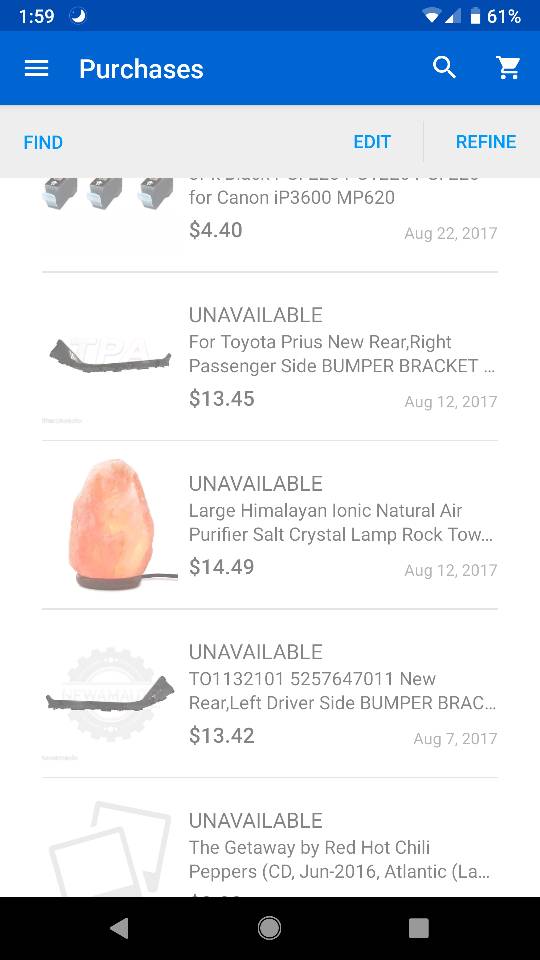This image displays a smartphone screen featuring a detailed overview of a shopping page. The header of the page has a blue background with white text. On the top left corner, there is a menu icon, followed by a "Purchase" option to its right. On the top right corner, two icons are visible: a search button and a cart icon, both in white. Just below these icons, there are buttons labeled "Edit" and "Refine" in blue, positioned on the top left. Beneath the menu icon, there is a "Find" option, also in blue.

Displayed below this header are five purchased products, with their descriptions and purchase details. The first product's description is partially hidden, but it shows a price of $4.40, purchased on August 22, 2017. The second product is marked as unavailable and is described as a "Toyota Prius New Rear Right Passenger Side Bumper Bracket," priced at $13.45 on August 2, 2017. The third product is a "Large Himalayan Ionic Natural Air Purifier Solid Crystal Lamp Rock," costing $14.49 on August 12, 2017. The fourth product is a "Rear Left Driver Side Bumper Bracket," priced at $13.42 on August 7, 2017. The last product is titled "The Getaway by Dread Hot Chilled Pepper City," but the price is not displayed.